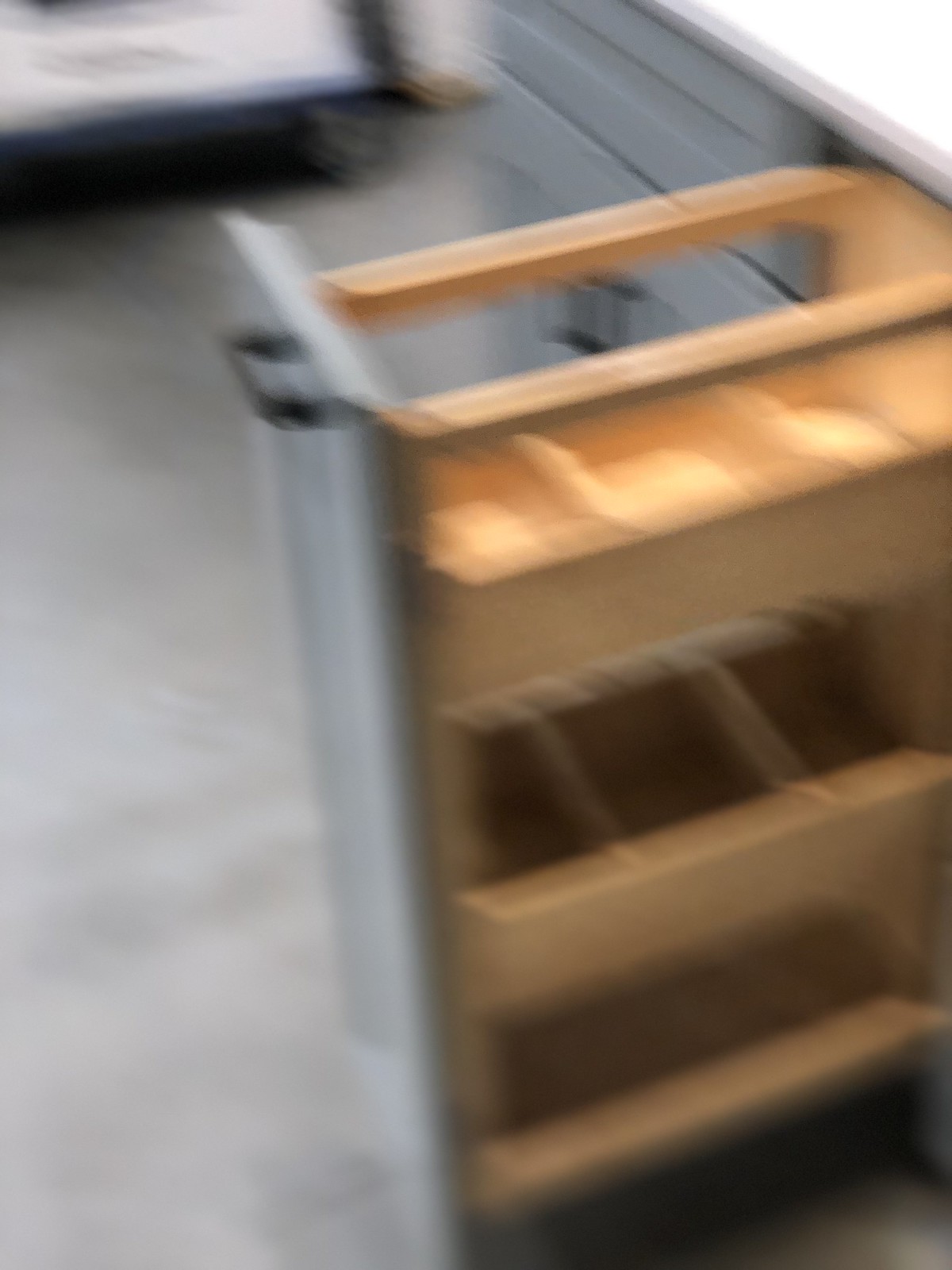In the image, a modern kitchen is depicted with a sleek, gray cabinet that features a unique pull-out mechanism. The cabinet has a single black handle that, when pulled, reveals three spacious, empty wooden drawers within. The surface of this cabinet appears to be crafted from pristine white granite, adding an element of elegance to the kitchen design. 

To the right of the open drawer, two additional handles are visible, suggesting the presence of more drawers within the cabinetry. The kitchen floor is a light gray, creating a clean and cohesive look with the overall color scheme of the room. 

Visible in the background is a white table, which has a distinctive black trim along its edges. The platform or base of the table is also white, complementing the minimalist and contemporary aesthetic of the kitchen.

This detailed caption gives a vivid portrayal of the modern, functional yet stylish design elements of the kitchen.